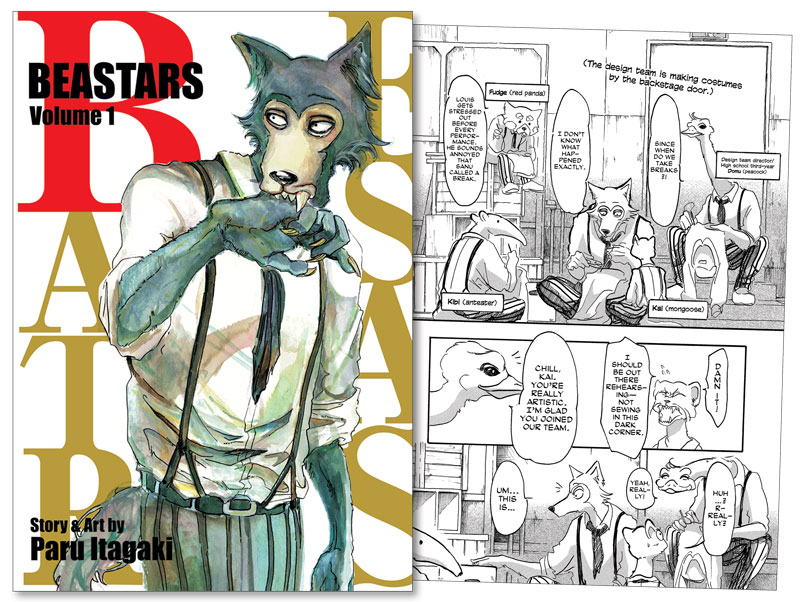This image is a combination showcasing both the front cover and two internal black-and-white panels of the manga "Beastars Volume 1," created by Paru Itagaki. The cover prominently features bold black text at the top announcing the title "Beastars" with "Volume 1" directly beneath it. The central figure is a wolf-like humanoid, evocative of a werewolf, dressed in a red dress shirt, pinstripe pants held up by suspenders, and a belt, with his necktie visible and his shirt sleeves rolled up. This character intensely bites his own hand while looking slightly to the left. 

Accompanying the cover are two black-and-white comic panels that depict a world populated by various anthropomorphic animals. These panels show a dynamic scene of different humanoid animals, including but not limited to a wolf, an ostrich with a human body, and an anteater, engaging in conversation and daily activities. Speech bubbles within the panels include dialogues such as, "The design team is making costumes by the backstage door," and, "Lewis gets stretched out before every performance. He sounds annoyed that Sanu called a break." Characters mentioned in the text include a red panda named Fudge, an anteater named Kibi, a mongoose named Cow, and another character named Kai being complimented on their artistic talent. Additionally, there are expressions of frustration and dialogue about rehearsing and sewing, adding to the vivid depiction of the characters' interactions and the world they inhabit.